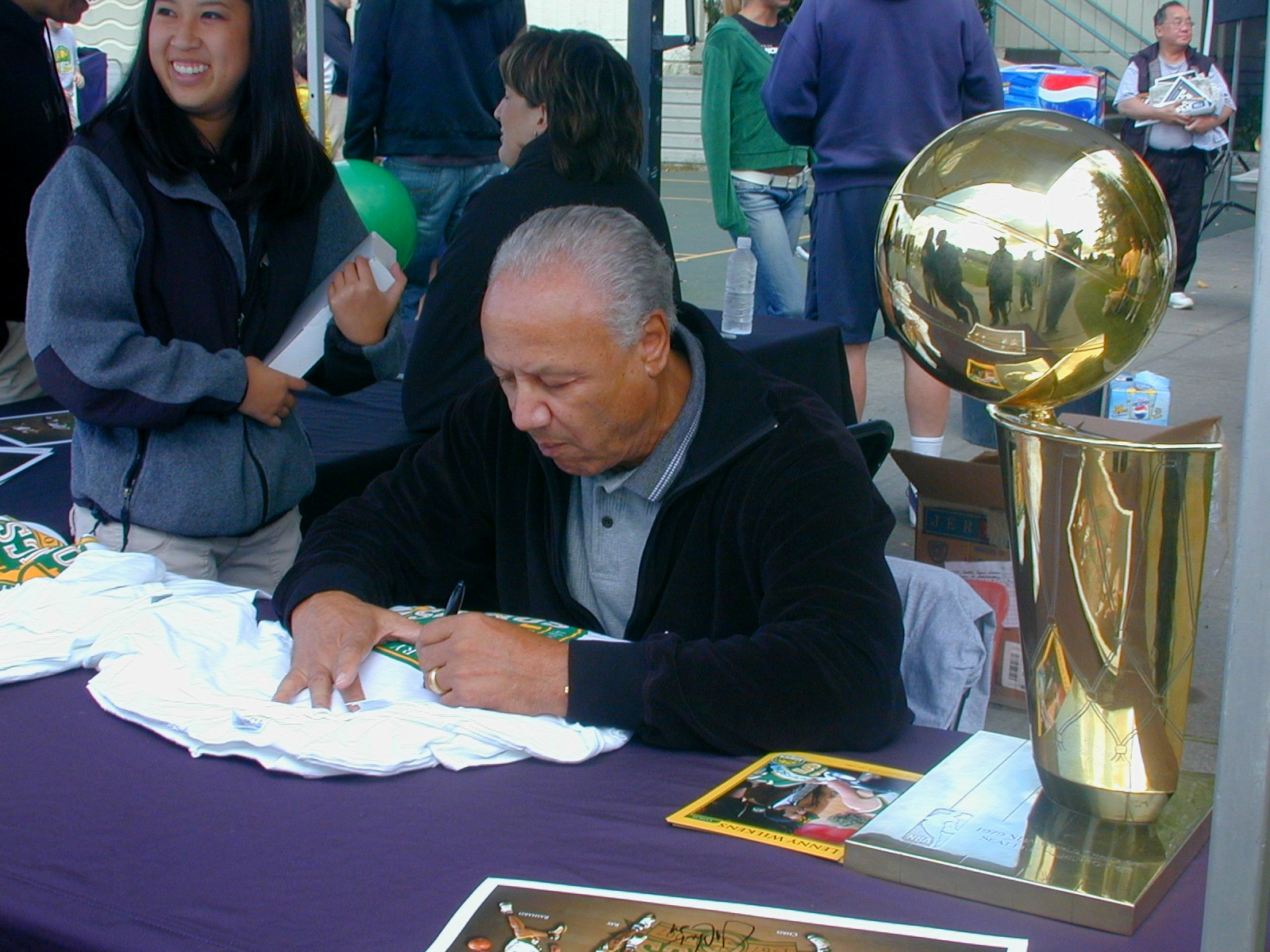In this outdoor color photograph, a mature gentleman, around 60 years old with gray and white hair, is seated at a table signing a white t-shirt. He is dressed in a black zip-up cardigan over a gray collared shirt. The table, adorned with a purple tablecloth, features several autographed photos and a very large golden trophy resembling a basketball, indicating his association with the NBA. To his left, a smiling young lady, possibly waiting for the signed t-shirt, adds to the lively atmosphere. In the background, set against an asphalt lot with yellow line markings, other people can be seen standing, talking, and smiling, contributing to the event's bustling ambiance. For more information, visit www.FEMA.gov.